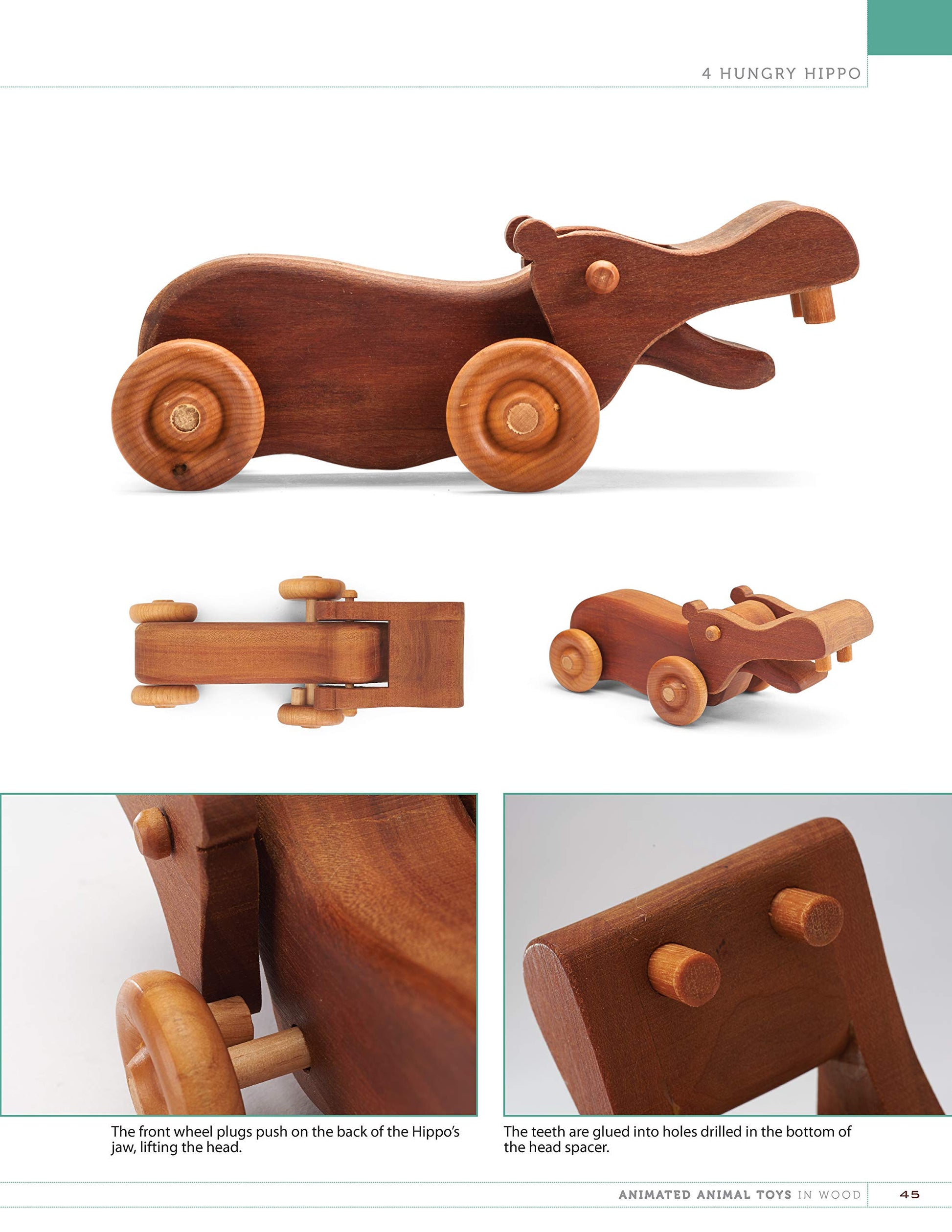The image appears to be a detailed page from a book or catalog, specifically showcasing a wooden hippo toy with wheels. At the top of the page, a green line leads to a green rectangle, next to which is the label "4. Hungry Hippo." Below this title, the page presents five distinct images of the toy, illustrating various angles and construction details. The primary image provides a profile view of the hippo toy, highlighting its open mouth, wooden dowel teeth, ears, eye, and lighter brown wheels, complete with a notable black spot on the rear left wheel.

Further images include a top-down and side view, offering a comprehensive look at the toy's shape, wheel placement, and head construction. There’s also a close-up from underneath, showcasing the toy’s base and connection pieces. Additionally, the page provides detailed views of the teeth and wheel mechanisms, explaining how the front wheel prongs push on the back of the hippo's jaw, lifting its head. The teeth are described as being glued into holes drilled in the bottom of the head spacers. Finally, at the bottom right corner of the page, the title "Animated Animal Toys in Wood" and the page number "45" are displayed, indicating the source of this detailed description. The overall color scheme of the hippo toy is a reddish-brown hue.